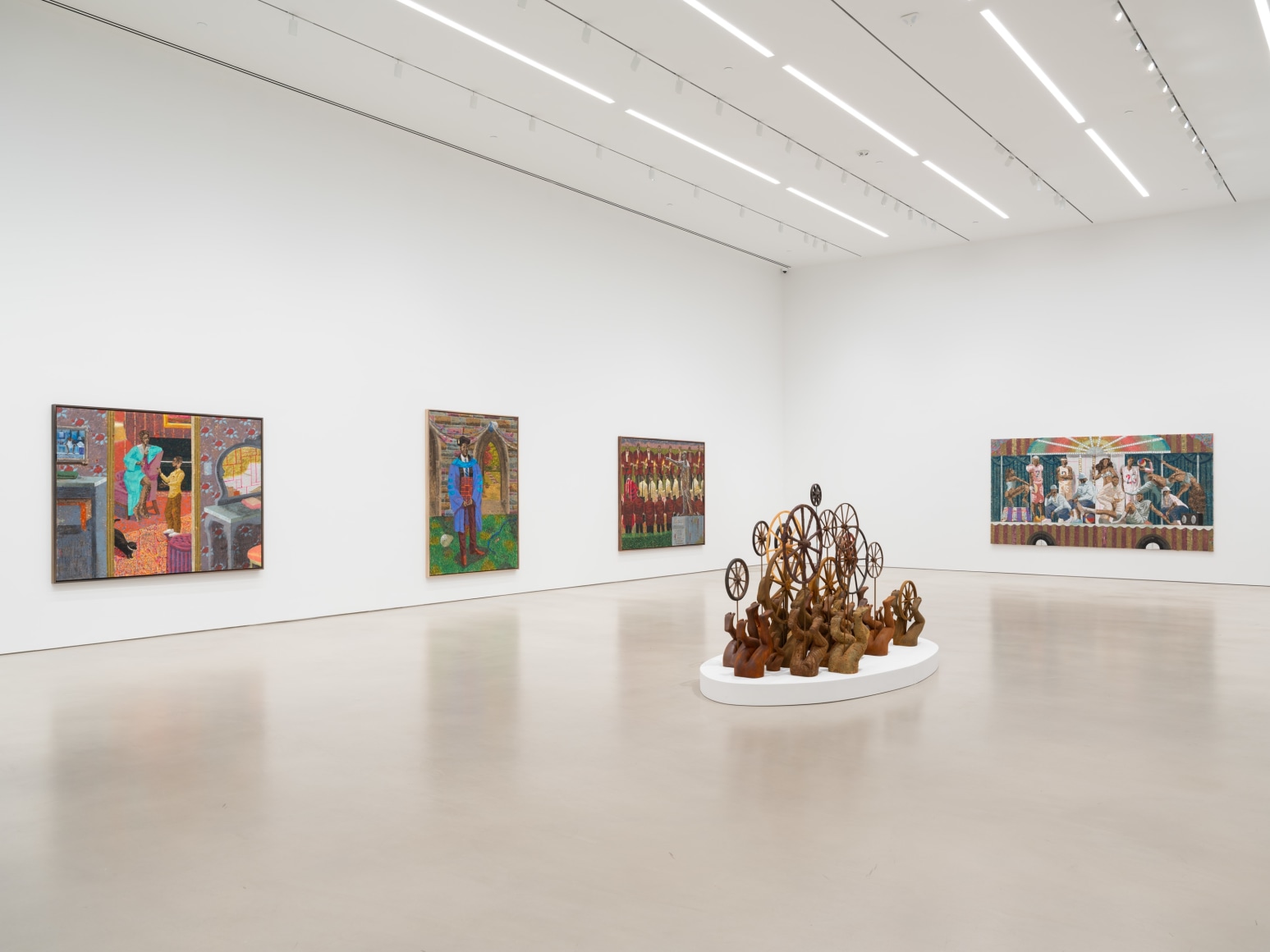This is a detailed color photograph of the interior of a contemporary art gallery. The setting is minimalist with white walls and ceiling, accentuated by slick, shiny white concrete floors that reflect the shadows of the artworks. Illuminated by strips of white overhead lights, the gallery houses four large, vibrant paintings in a spectrum of colors, each an abstract composition.

On the left wall, there are three paintings, starting with one showcasing a person in a blue dress sitting in a chair, while another individual in a yellow shirt and brown pants stands nearby. The second painting depicts a person in a blue graduation-style gown with brown pants standing next to an arch. The third artwork displays rows of indistinct figures clad in red and white attire. The right wall hosts a single large rectangular painting, featuring a dynamic, semi-blurred scene of various athletes.

Dominating the center of the gallery is a striking brown sculpture set on a white oval base. This kinetic piece portrays upside-down legs in pedaling positions, with wheels of different shapes and sizes suspended above them, evoking the motion of cycling. The entire installation creates a vivid and engaging visual experience within the pristine gallery space.